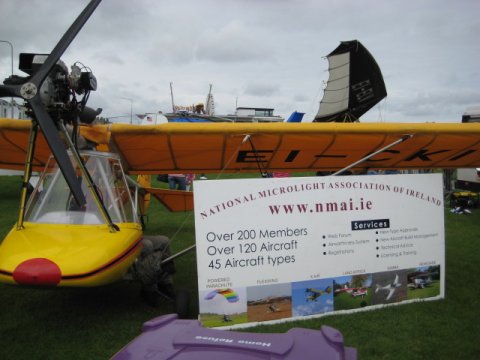This outdoor photograph captures a get-together for the National Microlight Association of Ireland under a gray, cloud-filled sky. Dominating the left side of the image, a single-engine plane features a cockpit with a black engine adorned in yellow and red hues, marked with the text "EI-CKI" beneath its yellow and red wing. A separate wing stands out in the distant top right. The bottom half of the background is a lush green field. In the bottom right corner sits a colorful sign in purple, white, red, black, blue, and green. The sign details the National Microlight Association of Ireland, www.nmai.ie, boasting over 200 members, 120 aircraft, and 45 aircraft types, with smaller text about services that is too blurred to read.